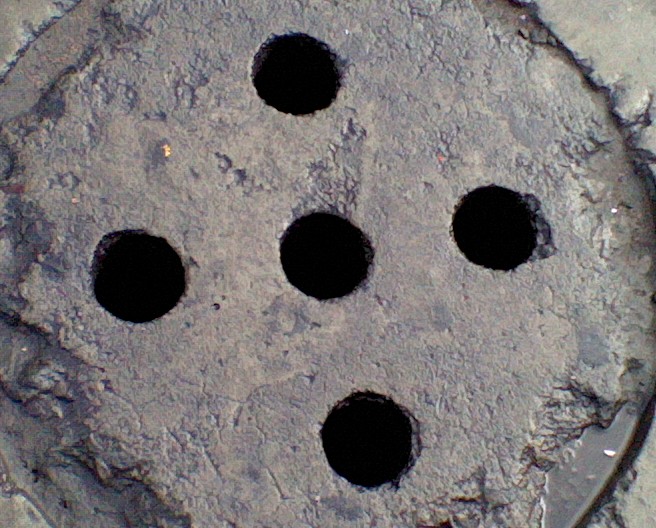This black-and-white photograph captures an extreme close-up of a rugged, round object, possibly made of cement, stone, or metal. The circular item features five distinct black holes arranged like the face of a die, with one hole in the center and one at each of the cardinal points—north, south, east, and west. The surface of the object is rough and cracked, with varying levels creating a slightly elevated platform around the edges. Flecks of yellow and reddish-orange are visible amidst the textured, predominantly gray and brown surface. The entirety of the photograph is filled by this enigmatic object, which is framed by additional roughness extending to the edges, reinforcing the mysterious, multi-layered appearance of the item. The nature of the object remains uncertain, resembling either an unusual button, a drain, or perhaps some form of manhole cover.